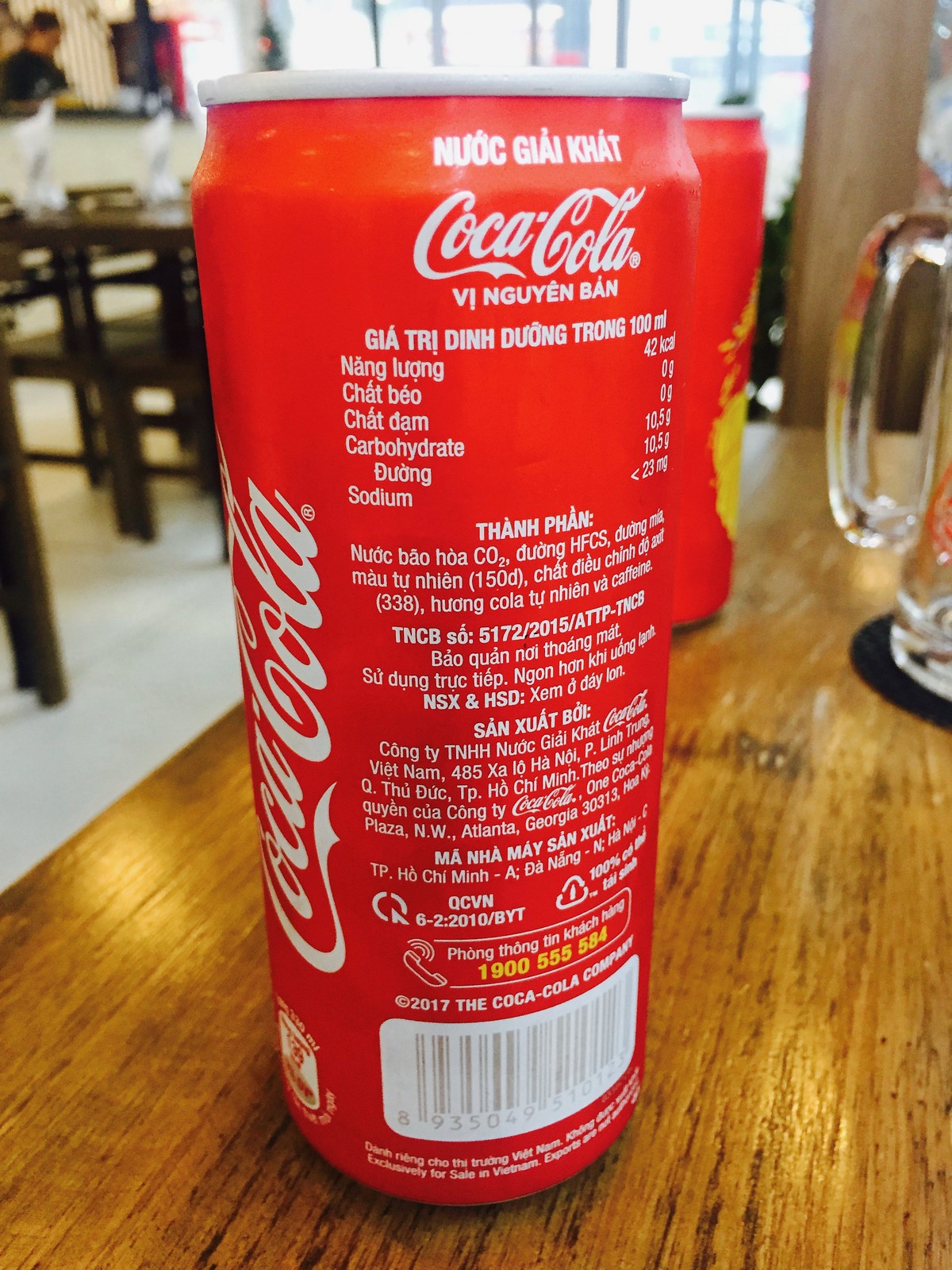In the image, there is a tall, red can of Coca-Cola prominently displayed on a wooden table, positioned towards the front center of the frame. The can, which is in Vietnamese, features the familiar Coca-Cola logo in white cursive text running vertically along the left side with additional white lettering across the top stating "NƯỚC GIẢI KHÁT." On the back of the can, visible details include nutritional information listing 42 calories per 100 milliliters and 10.5 grams of carbohydrates. Below the logo, further text outlines the ingredients and includes a barcode and a customer service number. A QR code is situated at the bottom right of the can.

Behind the main can on the right, there is a partial view of another red Coca-Cola can with a hint of yellow along its edges. Also visible in the same background area is the handle and bottom of a clear beer mug resting on a black coaster. The setting appears to be an indoor restaurant with a gray floor and several brown tables equipped with napkins and occupied by patrons. A window at the top of the frame allows natural light to illuminate the scene.